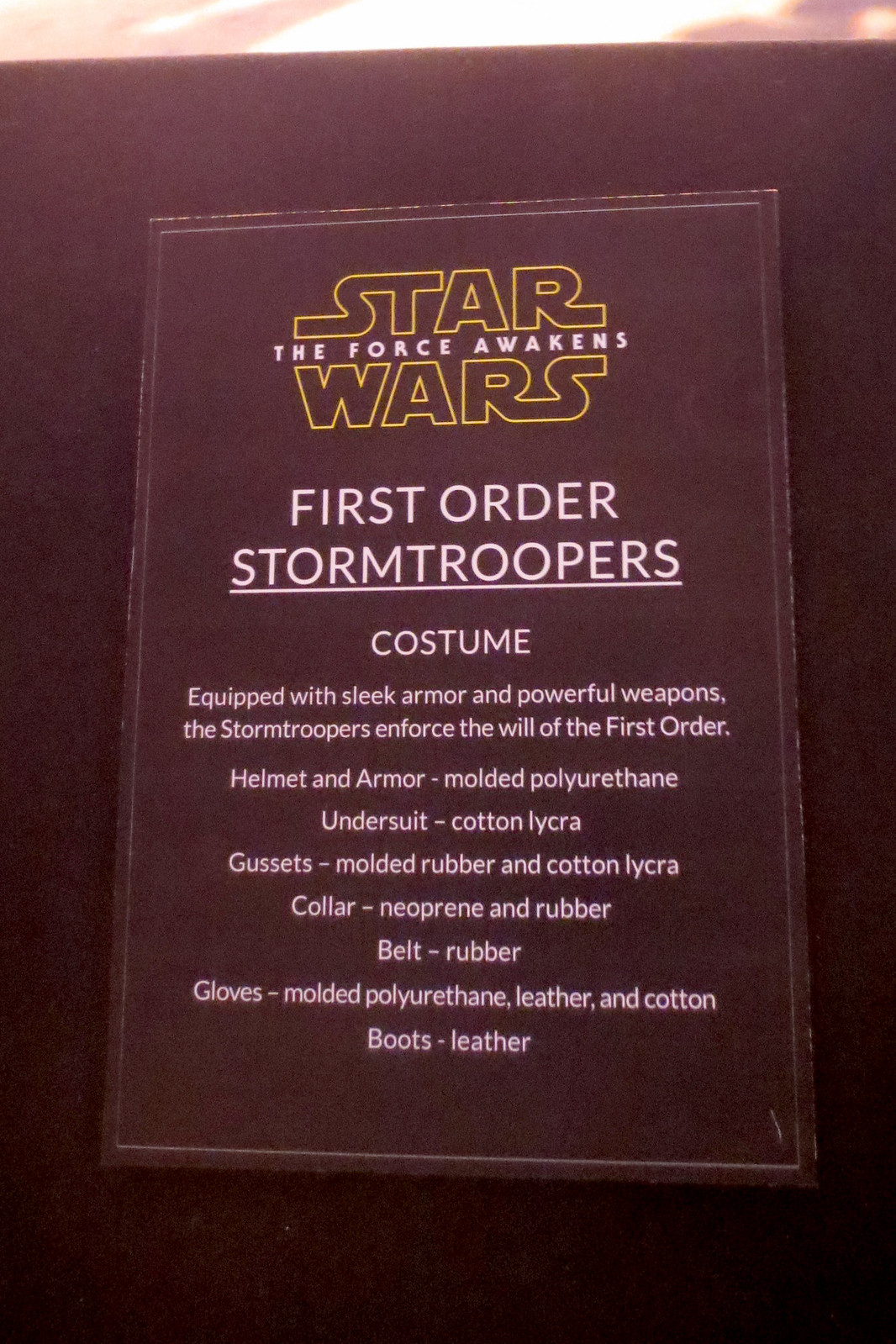This image depicts a close-up photograph of an informational placard against a solid black or dark maroon wall. The placard itself is a black rectangle with a thin white border. At the very top, in black text with a yellow outline, it reads "Star Wars," and between the words "Star" and "Wars," in white text, it says "The Force Awakens." Below this title, the card details the costume elements of the First Order Stormtroopers from the movie. The text reads: "First Order Stormtroopers. Costume. Equipped with sleek armor and powerful weapons, Stormtroopers enforce the will of the First Order." The placard then lists the materials used for different parts of the costume: 

- Helmet and armor: Molded polyurethane 
- Undersuit: Cotton lycra 
- Gussets: Molded rubber and cotton lycra 
- Collar: Neoprene and rubber 
- Belt: Rubber 
- Gloves: Molded polyurethane 
- Leather and cotton boots: Leather 

This plaque likely serves as an explanatory note for a display or exhibit featuring a First Order Stormtrooper costume from "Star Wars: The Force Awakens," detailing the construction and materials of the iconic armor.